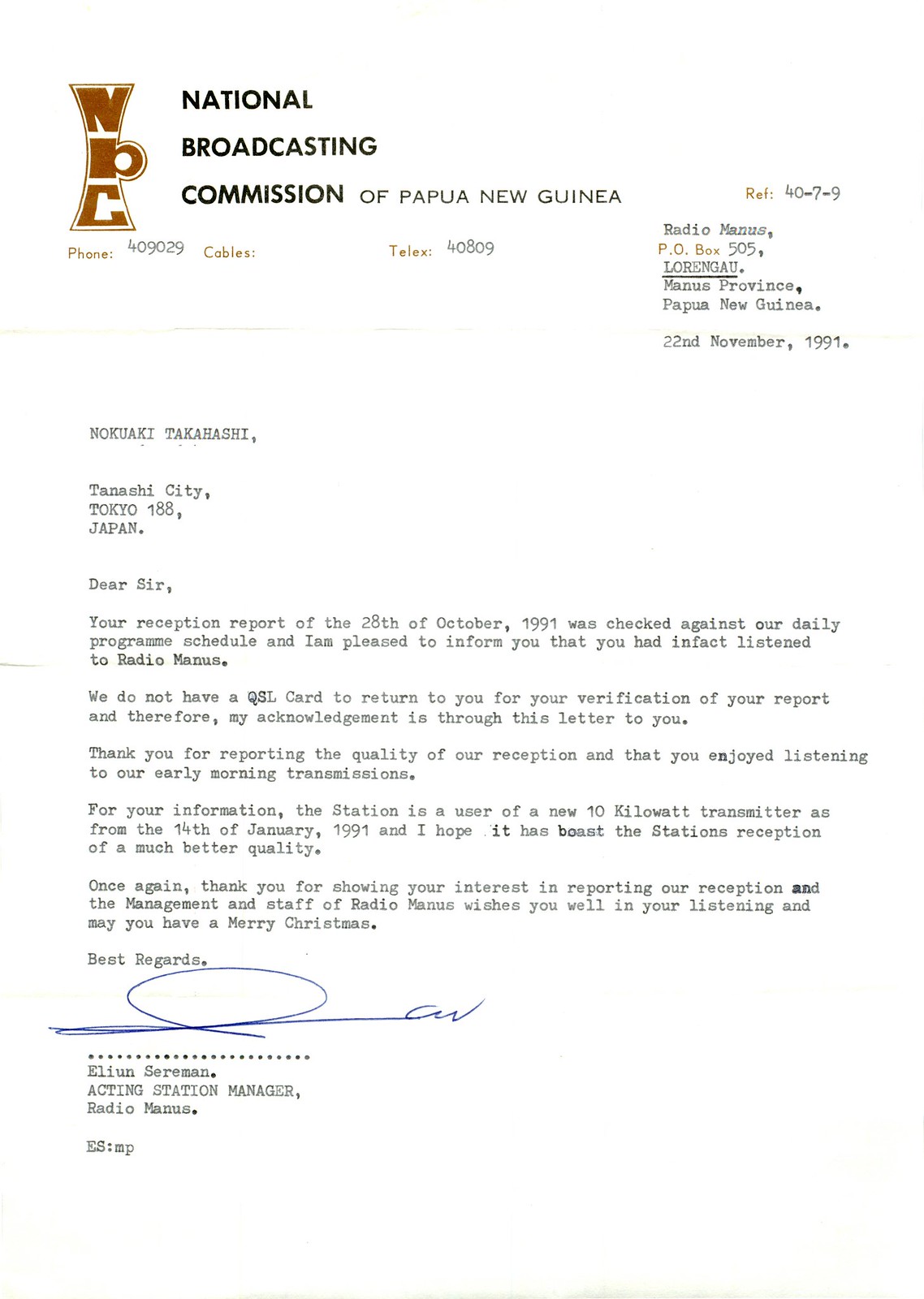This image showcases a printed letter on official stationery from the National Broadcasting Commission of Papua New Guinea. In the top left corner, there is a logo in a reddish-brown color, featuring the initials "NBC." Adjacent to the logo, in black text, it reads "National Broadcasting Commission of Papua New Guinea," followed by the organization's phone number, telex number, and address.

The body of the letter addresses Nukai Takashi in Tanoshi City, Tokyo, Japan, and is dated October 28, 1991. The letter confirms the reception of Takashi's report on listening to Radio Manus. It mentions that while there is no QSL card available to verify the report, this letter serves as formal acknowledgement. The letter continues by expressing gratitude for Takashi's feedback on the broadcast quality and mentions that the station has been using a new 10-kilowatt transmitter since January 14, 1991, which is expected to enhance reception quality.

The letter extends best wishes from the management and staff of Radio Manus, wishing Takashi a Merry Christmas. The letter is signed in blue ink by Eliam Searman, the Acting Station Manager of Radio Manus.